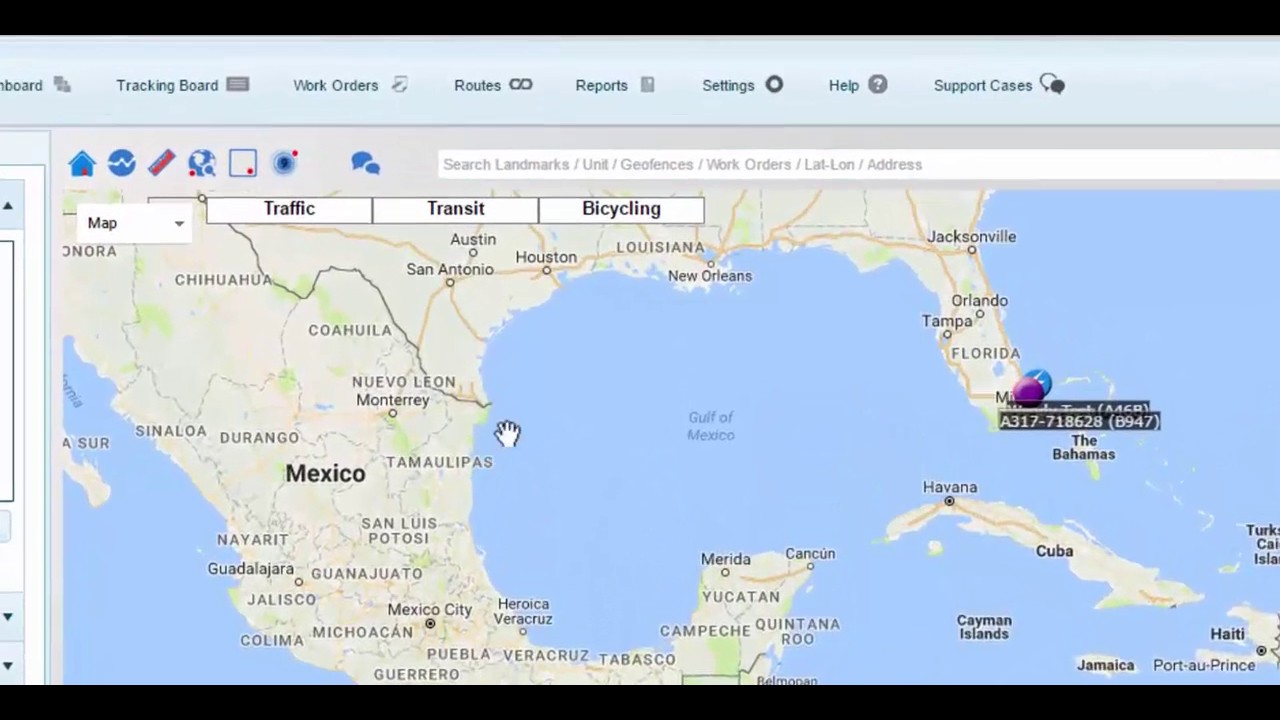The image depicts a screenshot of a website with a layout that is twice as wide as it is tall. The top 5% and bottom 5% of the image are framed by a black bar, creating a letterbox effect. Below the top black bar, there is a classic medium gray bar spanning horizontally for about 15% of the total height. This gray bar resembles the standard background color used in most web browsers, containing various navigational buttons labeled in black text. From left to right, the buttons are labeled: Dashboard, Tracking Board, Work Orders, Routes, Reports, Settings, Help, and Support Cases.

Dominating the main section of the image is a detailed map of the southern United States. The map extends from around two-thirds down Georgia to nearly the southern tip of Mexico, capturing regions including the southeastern U.S., Cuba in the lower right, and Mexico on the left. Florida is located towards the upper right of the map. On the map, there are several pins marking specific locations. Notably, in southern Florida, there is a purple pin on the lower right and a blue pin just below it. Each pin is accompanied by alphanumeric labels that appear to be randomly assigned.